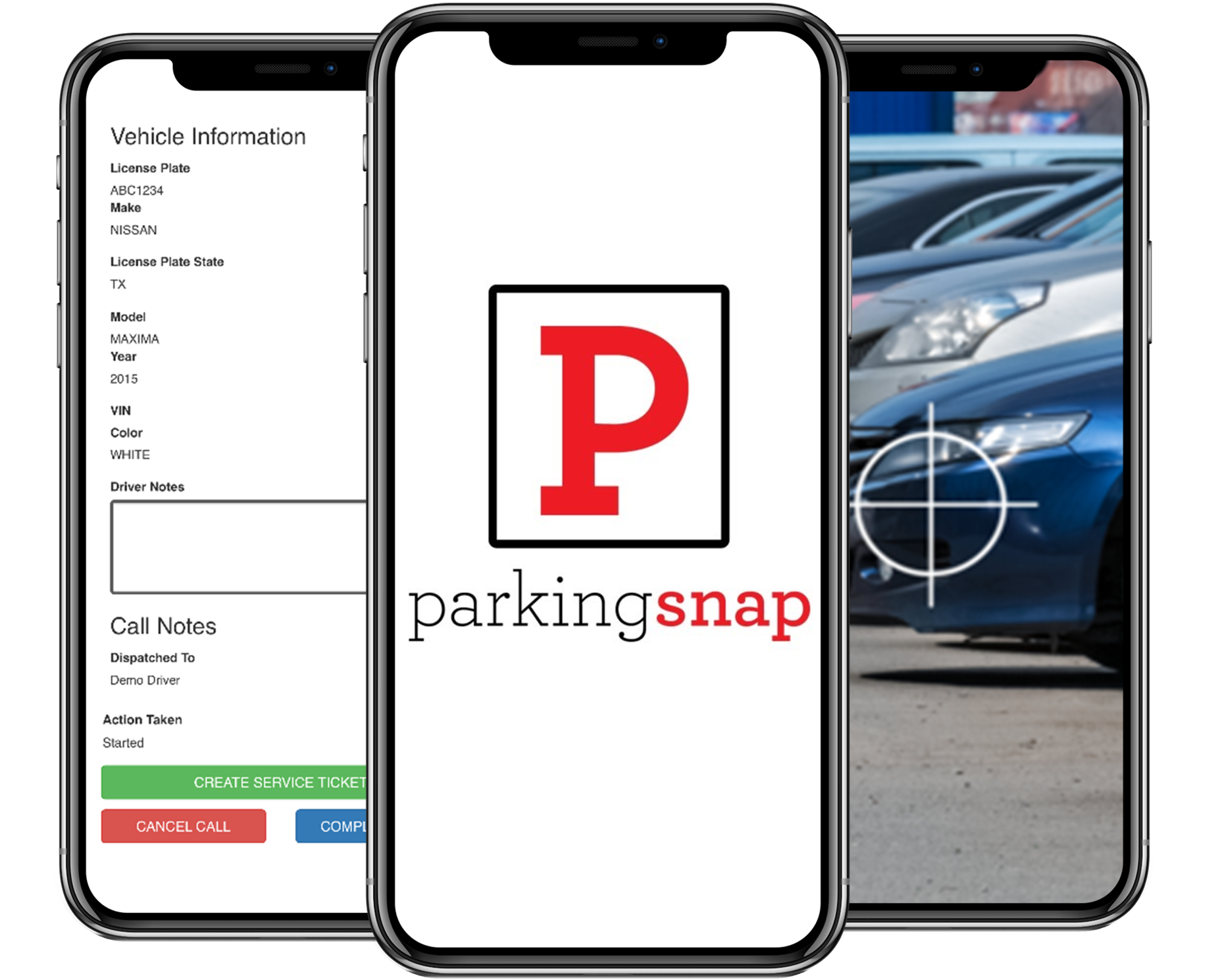The image is a screenshot featuring three mobile phones arranged in a row. The first two phones are positioned in the background, while the center phone is forward-facing.

**Phone on the Left:**
The display on the left phone shows detailed vehicle information. Below the header "Vehicle Information," various specifics are listed: 
- **License Plate:** Texas 
- **Make:** Nissan 
- **Model:** Maxima 
- **Year:** 2015 
- **Color:** White 
Notably, the VIN (Vehicle Identification Number) is absent. There are sections for "Driver Notes" and "Call Note." Additionally, "Dispatch to Demo Driver" and "Action Taken: Started" appear on the screen. At the bottom, there are three color-coded action buttons:
- **Green Button:** "Create Service Ticket"
- **Red Button (left):** "Cancel Call"
- **Blue Button (right):** The text is unreadable.

**Phone in the Center:**
The middle phone's screen features a white background dominated by a logo: a red 'P' enclosed in a black-outlined box. Below the logo, the name "ParkingSnap" appears, with "parking" in black and "snap" in red, all in lowercase. The screen also displays an image of cars parked in a parking lot, with one vehicle highlighted by a target icon.

The third phone on the right is hidden, providing no visible information. The carefully arranged composition and highly detailed interfaces suggest a focus on vehicle management and parking solutions.